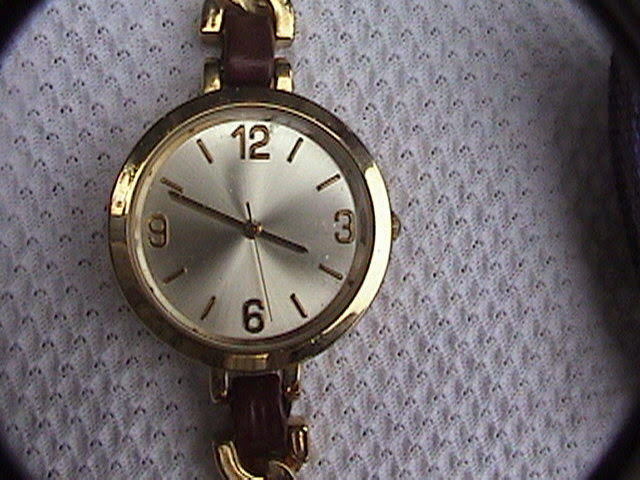This image features an elegant wristwatch placed on a white, textured cloth. The watch boasts a lustrous gold bezel and a matching gold strap, creating a striking contrast against its polished silver dial. The face of the watch is minimalist, displaying only the numbers 12, 3, 6, and 9, while the remaining hours are indicated by simple black lines. The time on the watch is set to 3:49, with the minute hand near the 10-minute mark and the second hand, a much thinner line, approaching the 6, marking almost 30 seconds. The watch lacks any additional text or logos. The absence of any human elements in the photograph makes it challenging to determine the exact size of the watch, though it is presumably designed to be worn on the wrist.